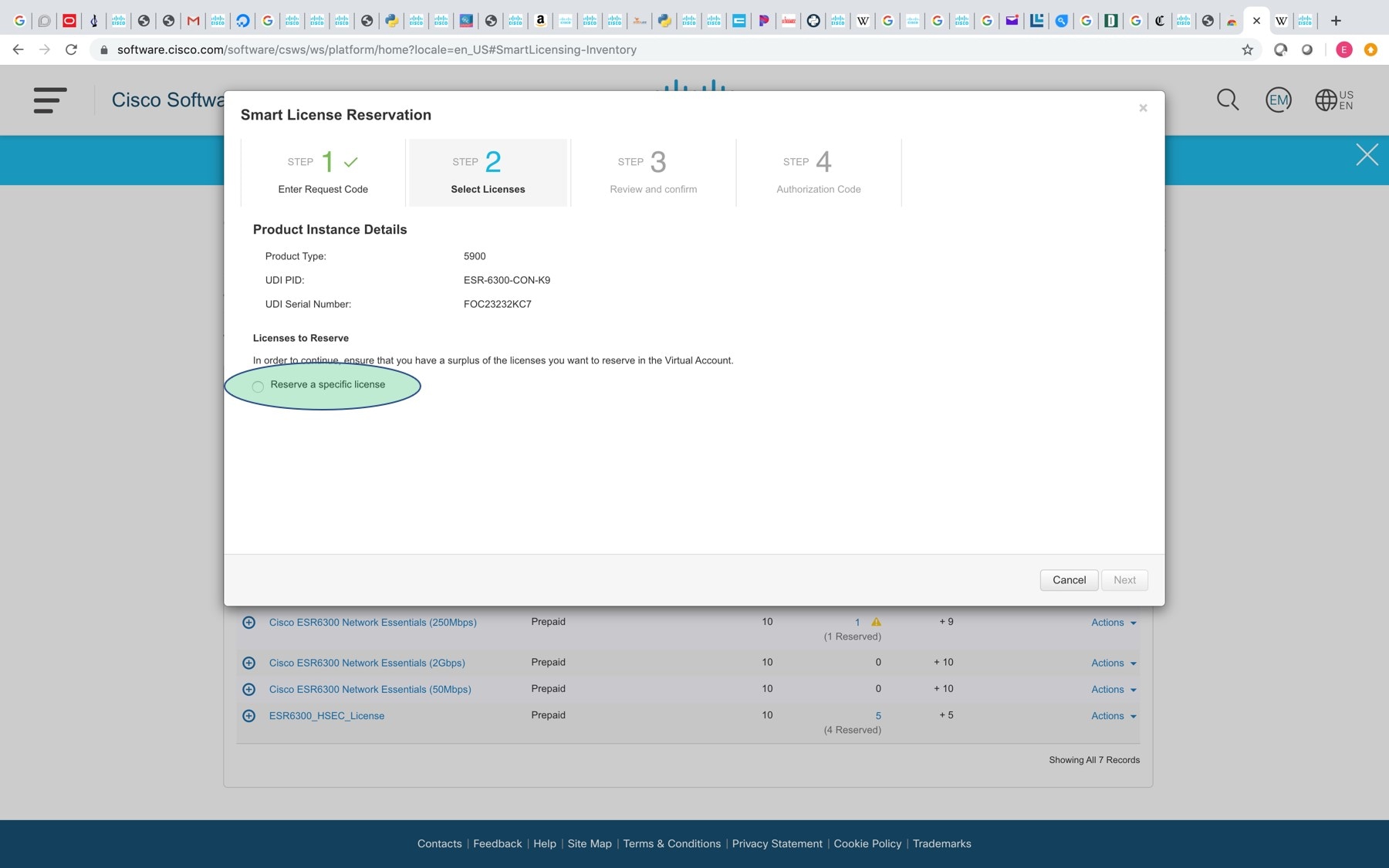The image showcases a screenshot of Cisco software, evidently from a web browser accessing software.cisco.com. The browser has an astounding 53 tabs open at the top. The software's interface displays the "Smart License Reservation" process, currently on step 2 of 4. In this step, the user is involved in selecting licenses, including product instance details and product type. One specific product, marked as ESR 54300CON-K9, is visible, though some information appears blurry. 

A highlighted circle draws attention to the "Reserve a specific license" option, which is not selected. The buttons "Cancel" and a grayed-out "Next" are located at the bottom right, suggesting that further selections are necessary to proceed. In the background, references to "Cisco Network Essentials" can be seen. 

Additionally, there are dropdown menus labeled "Actions," and at the bottom of the interface, several links are available, including "Contacts," "Feedback," "Help," "Sitemap," "Terms and Conditions," "Privacy Statement," "Cookie Policy," and "Trademarks."